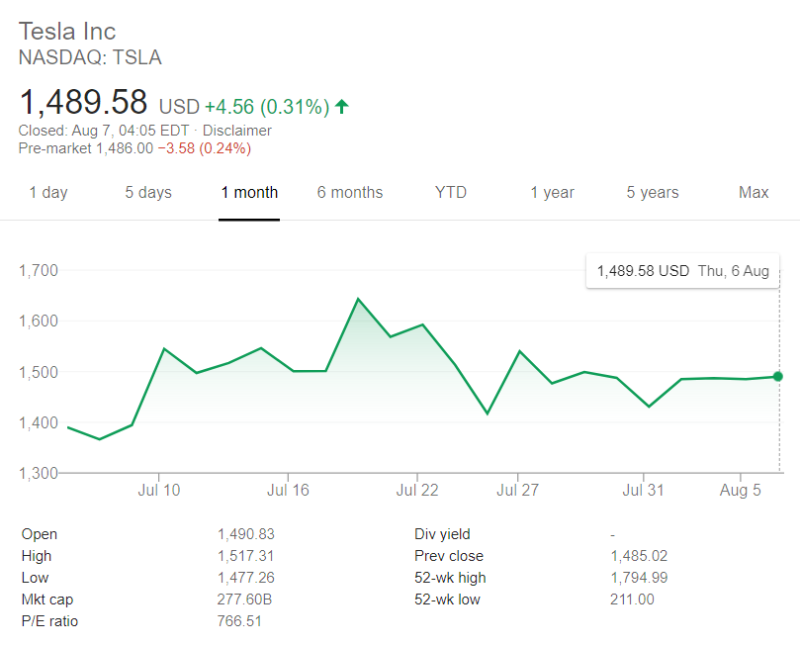This screenshot from the Nasdaq webpage showcases the current stock performance of Tesla (TSLA). At the precise moment captured, Tesla's stock price is $1,489.58 USD, experiencing an increase of $4.56 or 0.31%. The webpage features a graph on the bottom section, depicting the price movement with a green zigzag line that fluctuates, illustrating various plateaus and dips. The y-axis on the left side of the graph denotes price levels, marked at intervals of $1,700, $1,600, $1,500, $1,400, and $1,300. The x-axis at the bottom indicates dates, specifically highlighting July 10th, July 16th, July 22nd, July 27th, July 31st, and August 5th.

A white box within the graph indicates the current price and date: $1,489.58 USD on Thursday, August 6th. Additionally, the "1M" (one-month) chart view is selected, as highlighted by bold black text and an underline. Below the graph, detailed stock metrics are presented in two columns, covering: stock open, high, low, market cap, P.E. ratio, dividend yield, previous close, 52-week high, and 52-week low.